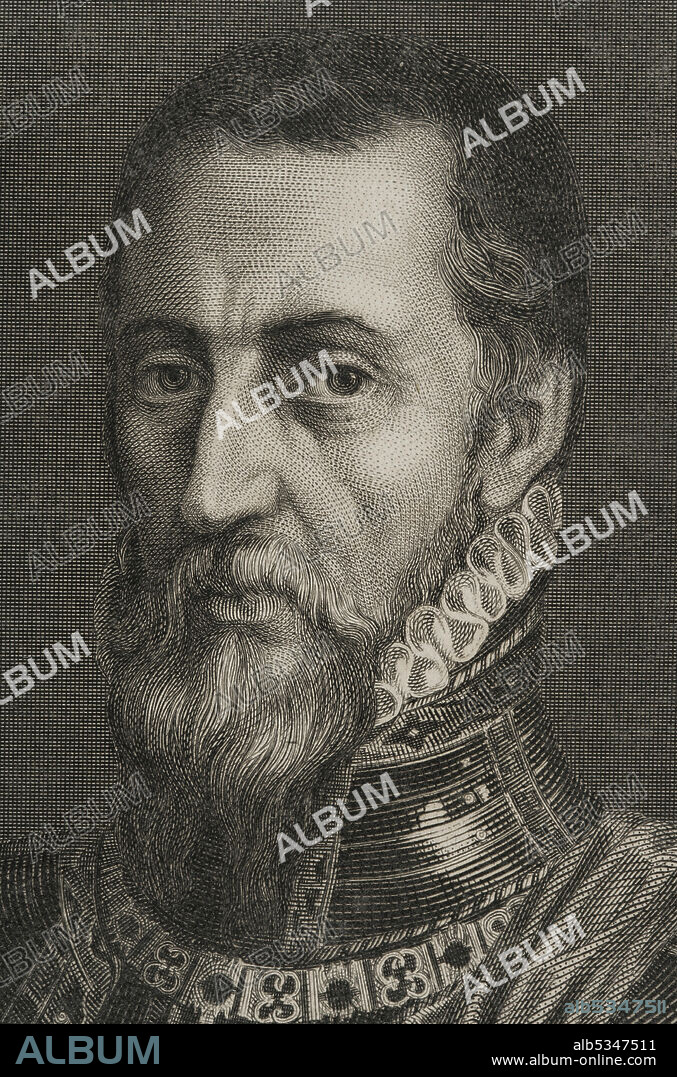The image depicts a detailed, albeit pixelated, black and white etching or sketch of a man, possibly from the Middle Ages or the Shakespearean/Victorian era, characterized by fine lines that resemble the texture of a dollar bill. The man appears to be a white male around his 50s, with short, dark hair, a beard, mustache, and sideburns extending to his ears. His expression is calm, and he has a long, slender nose with eyes that seem to look directly at the viewer. He's adorned in a white, ruffled collar typical of the era, sitting above a ribbed or armored neck piece with vertical strips and periodic etchings. Below this, the attire suggests further intricate designs—possibly another collar with four-leaf clover-like patterns and chain mail beneath. The entire vertical rectangular image is dominated by a watermark reading "ALBUM" at an approximately 40-degree angle, with additional small text at the bottom suggesting details like "ALBS" or possibly a URL.